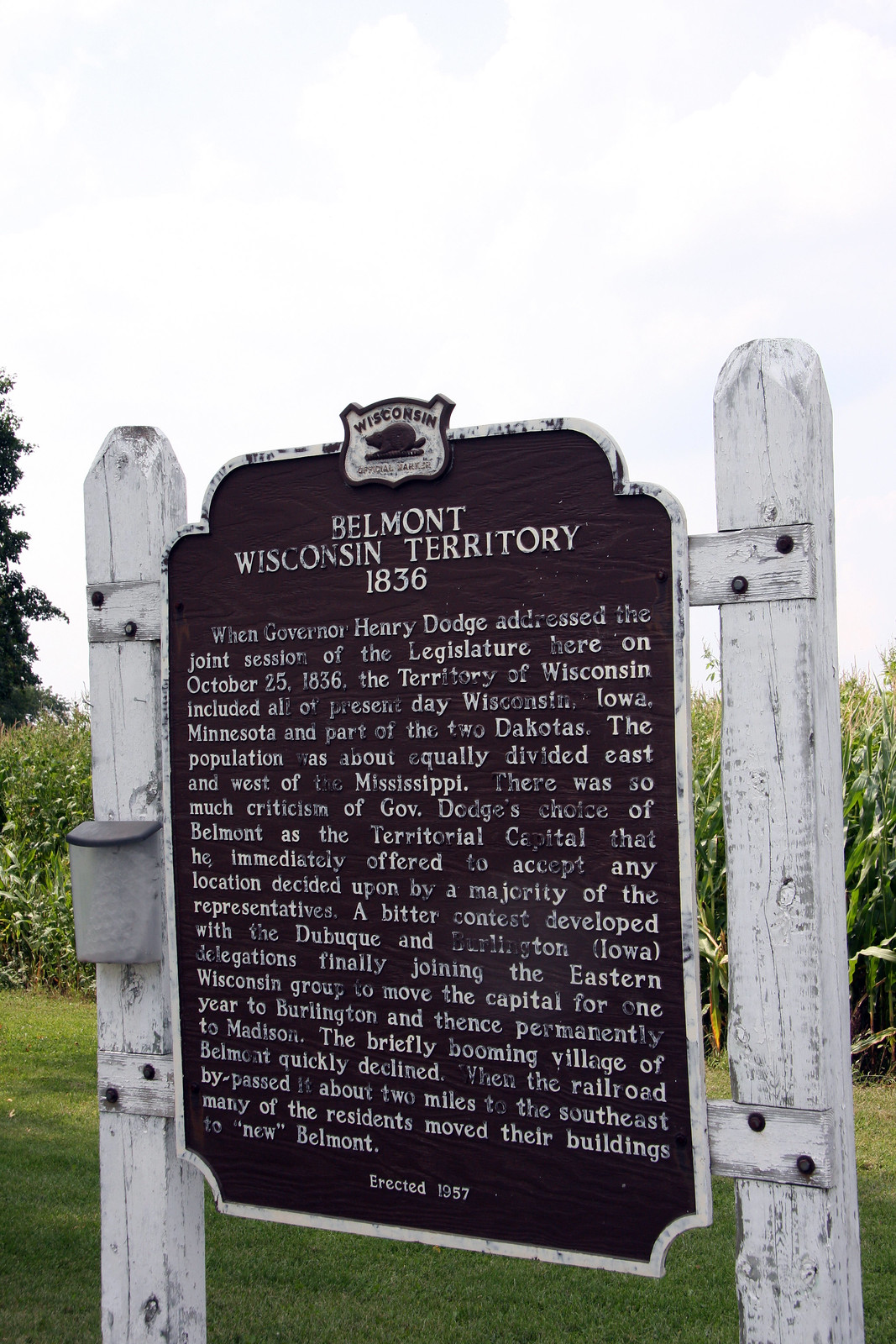The image depicts a state historical marker in Belmont, Wisconsin. The roughly rectangular marker, black with terraced and curved elements, features the Wisconsin state seal at the top, which consists of black text and a logo on a shield-shaped white background. The title "Belmont Wisconsin Territory 1836" is prominently displayed at the top, followed by detailed historical information in white text. It explains that on October 25, 1836, Governor Henry Dodge addressed the Wisconsin territorial legislature here; at that time, the Wisconsin Territory included all of present-day Wisconsin, Iowa, Minnesota, and parts of the Dakotas. Due to significant criticism over Belmont being chosen as the territorial capital, Dodge offered to accept any majority-decided location. As a result, a contest ensued, ultimately relocating the capital to Burlington for a year and then permanently to Madison. The village of Belmont declined quickly when the railroad bypassed it, leading many residents to relocate. The marker, erected in 1957, is mounted on a frame with two white posts connected by cross beams. The left post holds a waterproof container for information. The background showcases a grassy area with tall stalks, possibly a cornfield, under daylight.